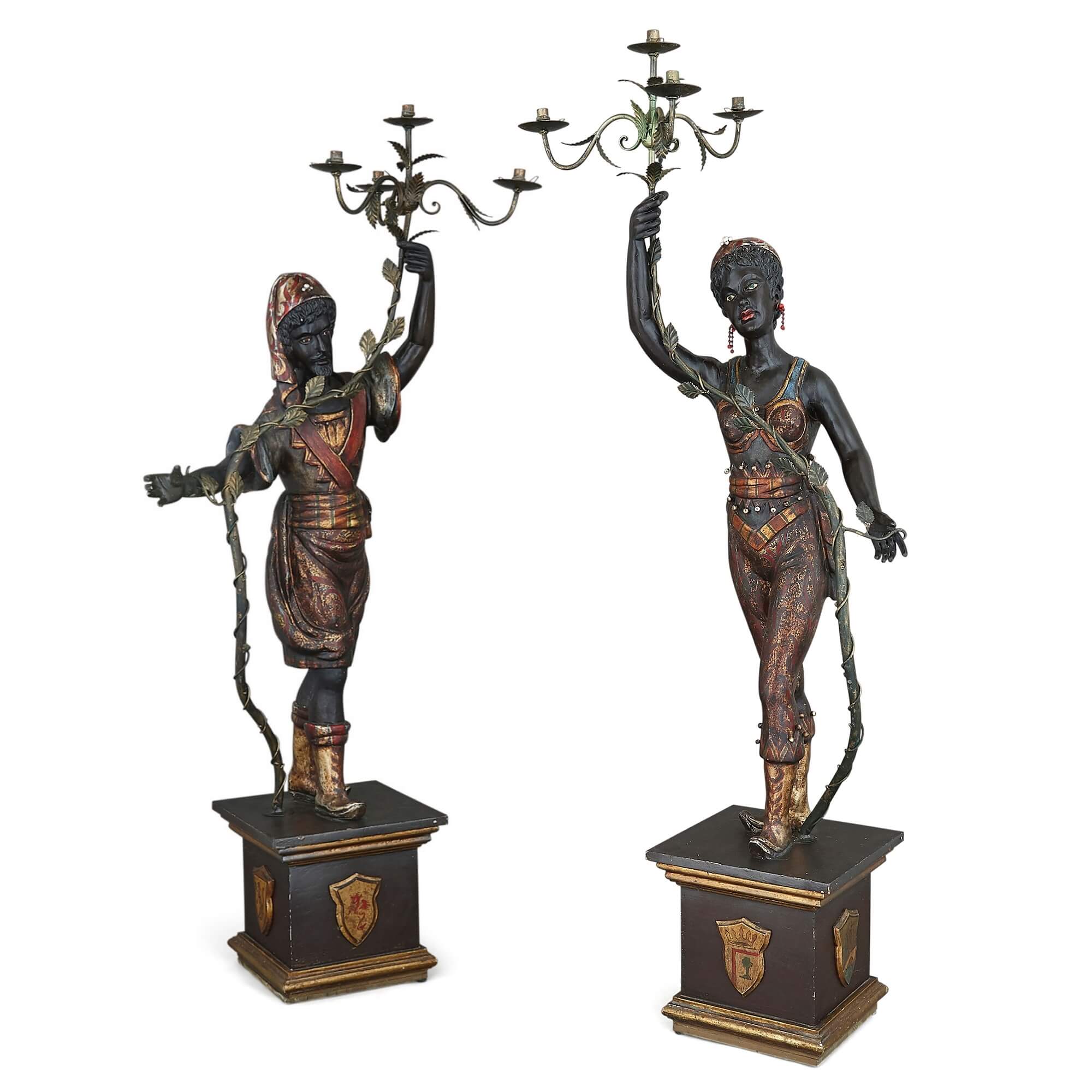This image features two ornate sculptures that function as dual-purpose candle holders. Each sculpture stands on a pedestal with bronze or brass rims and shield-like emblems on each of its four sides, forming a square base that appears to be gilded and rests on a wooden structure. The sculpture on the right portrays a woman adorned in a sleeveless top, pants, and boots, complemented by a belt around her waist. She holds a vine in her right hand that ascends gracefully to a candlestick-like lamp, suitable for multiple candles and featuring intricate leaf patterns. The sculpture on the left depicts a man wearing boots, shorts, a chest strap that resembles armor, and a headdress. He similarly grips a vine that stretches upward to support a candle holder. Both figures have a jet-black finish, enhancing their dramatic and somewhat tribal aesthetic, blended with designs that evoke ancient Greek or Roman styles. The meticulous detailing on these sculptures, coupled with their functional elegance, suggests a rich, historical inspiration fused with decorative artistry.